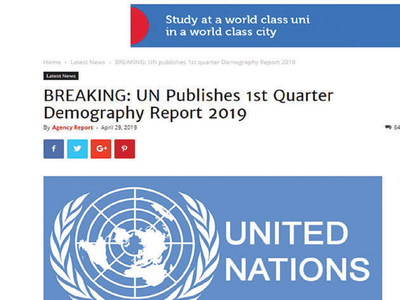This is a detailed screenshot featuring several distinct elements. At the top, there is a slate blue box containing promotional text that reads, "Study at a world-class university in a world-class city." Below this likely advertisement, there is a white background section displaying the title "Latest News" with a significant headline: "Breaking: UN publishes first quarter demography report 2019." This news article includes sharing options for Facebook, Twitter, Google+, and an unrecognized platform. As you continue to scroll down, another prominent blue box appears featuring the text "United Nations" alongside the distinctive United Nations emblem, which is characterized by a round design with olive branches encircling a world map.